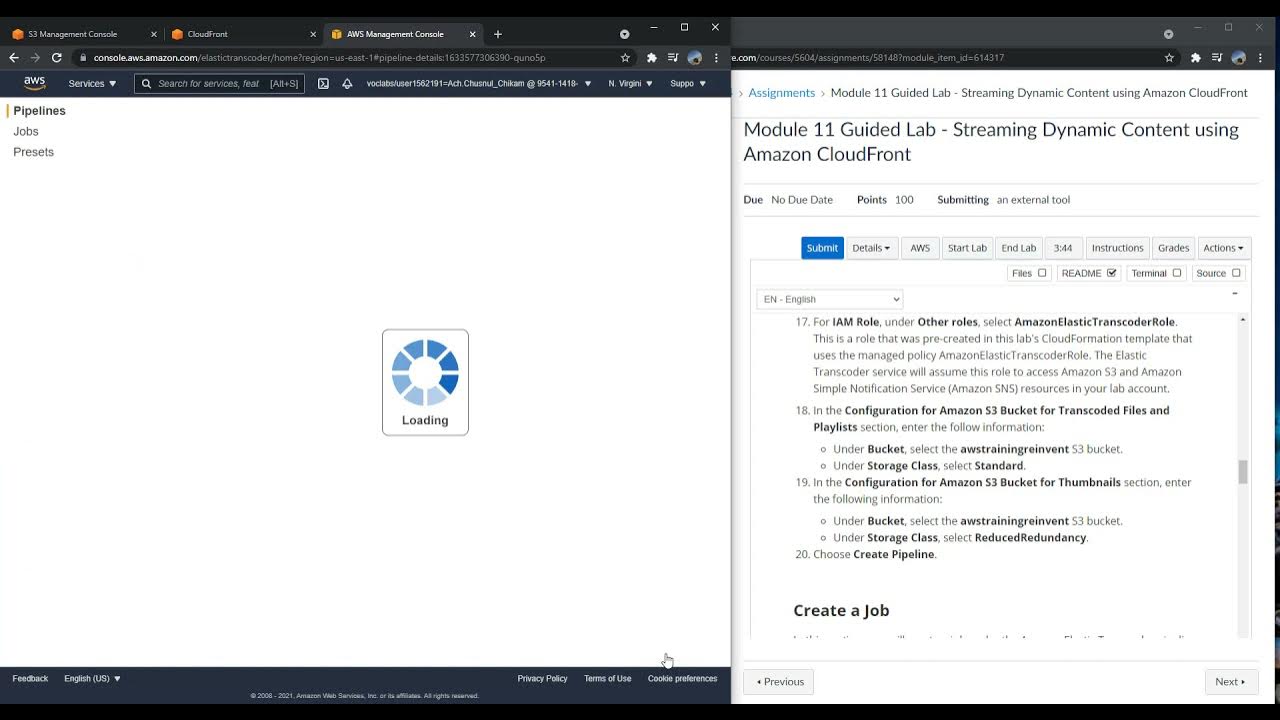This screenshot depicts a detailed view of a computer screen displaying elements from the AWS Management Console and accompanying instructional content. On the left, within the web browser with three open tabs, the active tab titled "AWS Management Console" is prominently featured. The interface includes black text labels such as "pipelines," "jobs," and "presets" against a white background. A distinctive blue circle indicates a loading screen with the text "loading."

To the right, the screen presents an educational module identified as "Module 11 Guided Lab: Streaming Dynamic Content Using Amazon CloudFront." This section lists items such as "assignments," "due," "no due date," "points 100," "submitting an external tool," and offers a variety of tabs like "Submit Details," "AWS," "Start Lab," and "Lab." Instructions within the module guide the user through various configurations, including setting roles for Amazon Elastic Transcoder and managing Amazon S3 bucket settings for transcoded files and thumbnails. The instructional text advises on selecting specific storage classes, entering required information, and creating pipelines and jobs within the AWS environment.